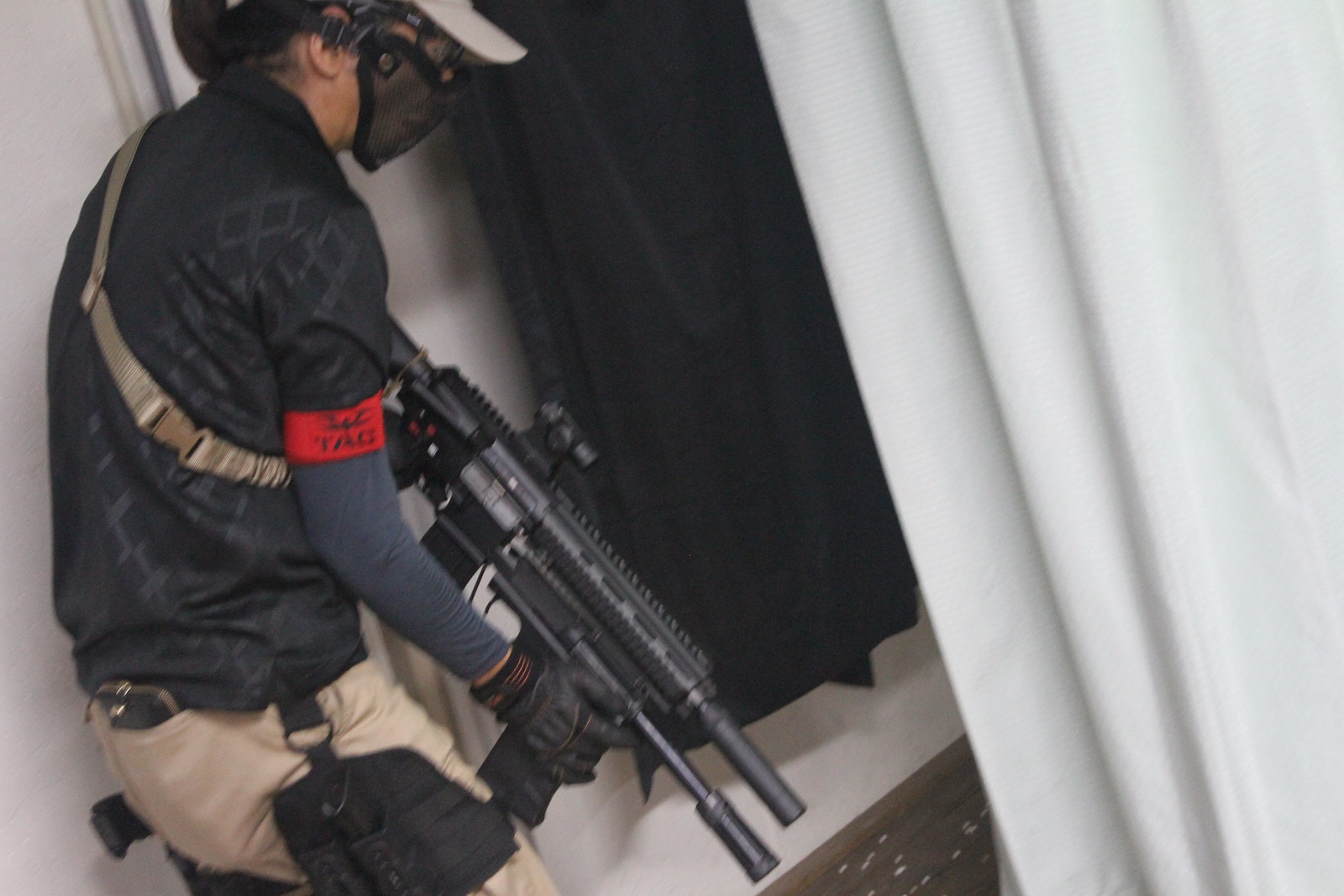In this photograph, a person appears to be in the midst of a training operation, possibly military or police. The individual is dressed in a black, long-sleeve shirt layered over a dark gray shirt, complemented by light tan khaki pants. The person has a tan hat, a full black face mask, clear goggles, and black gloves. Notably, a red armband is visible around the right upper arm. A pack attached to a tan strap is secured to their waist, with a black pouch hanging down their right thigh and a cell phone in their back right pocket. A secondary handgun handle is subtly visible behind their right hip.

The person is equipped with a large, black automatic weapon featuring two barrels and a possible scope, aimed downwards as they approach a curtained area. The weapon is held by a black-gloved hand gripping the handle, ready for action. They are entering an area delineated by a black curtain to the left and a white curtain to the right, with a darker brown floor. The scene is horizontal in orientation, capturing the person just as they lean against a white wall and step through the curtained entrance.